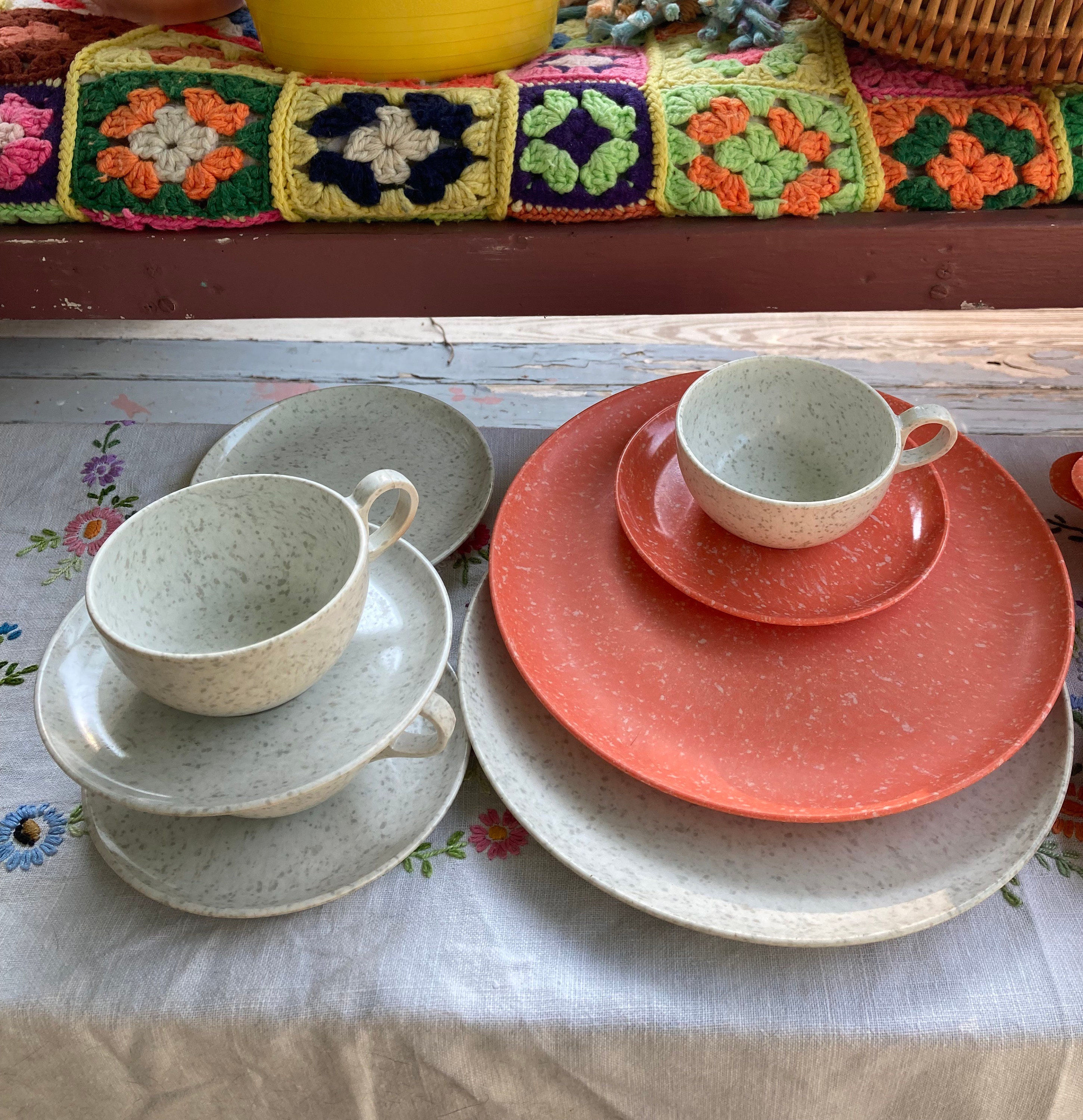This detailed image showcases an array of stone marble plates and cups meticulously arranged on a floral-patterned canvas tablecloth. At the forefront, in the lower part of the picture, a stack of plates and cups captures attention, featuring both white and red marbled pieces. The white marble items are speckled with dark gray, presenting a classic, stony aesthetic, while the red marble items are accented with white speckles, adding a vibrant contrast.

On the left side of the display, a series of plates and mugs are tiered—starting with a medium-sized plate at the bottom, followed by a coffee mug, then another plate, and a final mug crowning the stack. Behind these, a plate rests directly on the tablecloth's floral design, contributing to the visual interest.

The right side of the image highlights a larger plate with a white speckle pattern supporting coral-colored smaller plates, with a little saucer and another coffee mug perched neatly on top. 

The background provides a cozy context with a wooden bench draped with a quilt-like crocheted afghan adorned with colorful floral squares. A wicker basket peeks from the upper right corner, adding a rustic charm to the scene. The combination of the detailed table setting and the warm, textured backdrop creates an inviting and thoughtfully composed presentation.